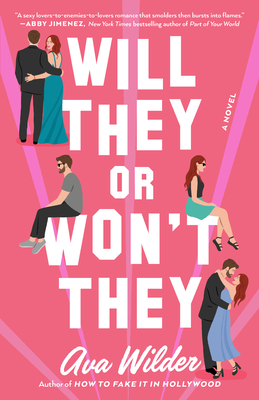The book cover features a vibrant pink background with light stripes radiating from the bottom to the top. Dominating the center in bold white capital letters is the title "WILL THEY OR WON'T THEY." At the top, in very small white print, there's a tagline including the words "a sexy lovers," though it's not fully legible. Above the title, in capital letters, is the name "Abby Jimenez." The detailed, colorful caricatures of couples are scattered throughout the cover. In the top left corner, a man and woman in formal wear, with the woman in a dark blue dress and the man in a dark suit, stand with their arms around each other, facing away but with the woman looking back towards the viewer. Sitting atop the word "WON'T," another couple faces opposite directions, the woman in a blue skirt and dark top, sporting dark glasses and long reddish-brown hair, and the man wearing a grey shirt and black slacks. In the bottom right corner, a dancing couple embraces; the woman in a long blue dress and the man in a black suit, depicted in a profile view. The bottom of the cover features the author’s name "Ava Wilder" in elegant cursive, followed by the subtitle in smaller white text, "Author of How to Fake It in Hollywood." The book's pink background is enhanced by light effects, giving it a vibrant, engaging appearance.